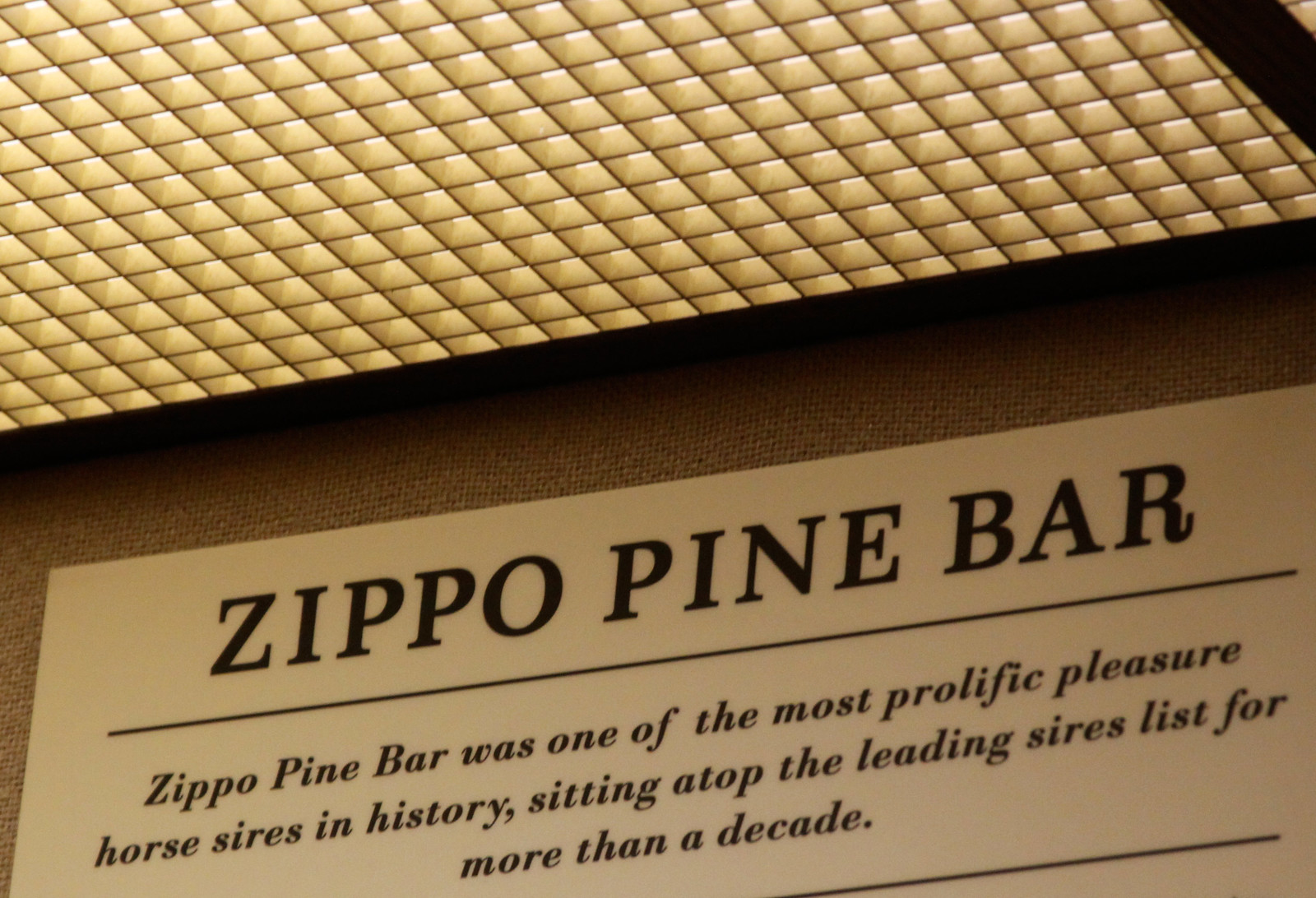The rectangular photograph was taken indoors against a backdrop of beige, almost tweed-like wallpaper or canvas. Dominating the upper portion of the image is a distinctive, grid-like drop ceiling from which small squares of light shine down, creating a golden yellowish glow. In the center of the image, prominently displayed on the wall, is a clean white sign with black lettering. The top portion of the sign boldly reads "Zippo Pine Bar," while a line below in smaller text states, "Zippo Pine Bar was one of the most prolific pleasure horse sires in history, sitting atop the leading sires list for more than a decade." The overall setting combines subtle textures and uniform lighting to emphasize the historical significance of Zippo Pine Bar.